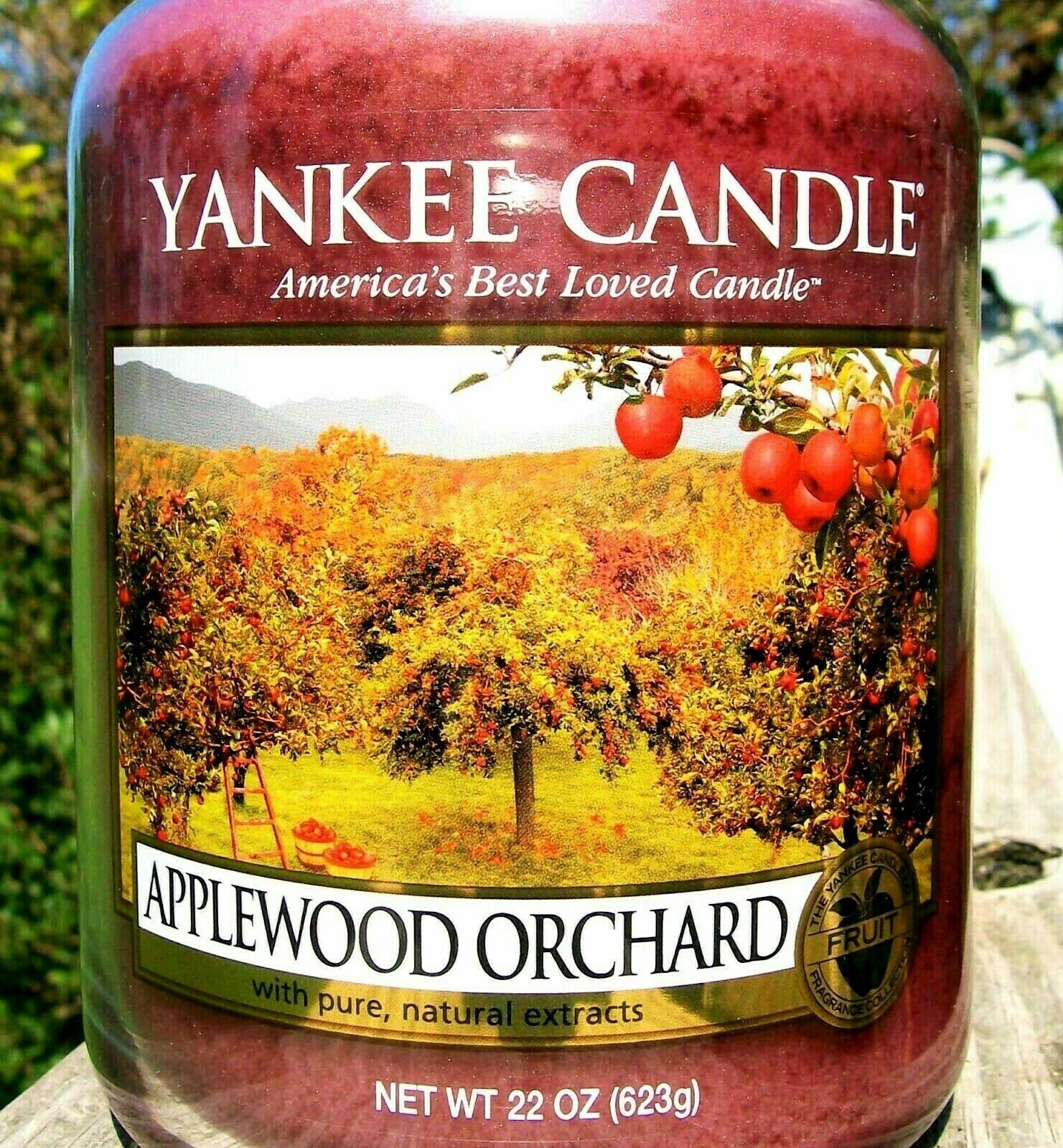This detailed image showcases a close-up of a bright red Yankee Candle encased in a glass jar, prominently displayed on a wooden table. The transparent label on the candle features the iconic "Yankee Candle" text in white at the top, followed by the phrase "America's Best Loved Candle" in smaller letters. The centerpiece of the label is a vivid photograph of an apple orchard, complete with apples hanging from tree branches visible in the top right corner. Below the image, a white banner reads "Applewood Orchard," accompanied by a gold round label inscribed with the word "Fruit." A gold banner beneath this declares "With Pure Natural Extracts." The candle's net weight is clearly marked at the bottom of the glass as 22 ounces (623 grams). The background of the photo is blurred, hinting at an outdoor setting with trees and foliage, though the primary focus remains sharply on the candle.